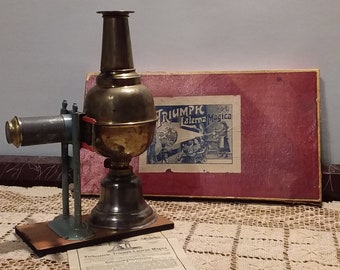This photograph captures a vintage scene, featuring an antique bronze object sitting on a tan, intricately designed knitted doily that covers a wooden table or shelf. The bronze artifact, with a bell-shaped base and an elongated cylindrical structure topped by a chimney, includes an additional side cylinder supported by a small green metal piece. In the background, there's an old photograph depicting a lady wearing an apron, seemingly in a kitchen setting, possibly attending to a fire. Accompanying the antique piece is a certification beneath it, although its details remain indiscernible. The scene is framed by a red box in the background, containing text that reads something akin to "Triumph Latte Magica," suggestive of a historical or magical relevance. The overall ambiance conveys a sense of historical intrigue, blending domestic and arcane elements.